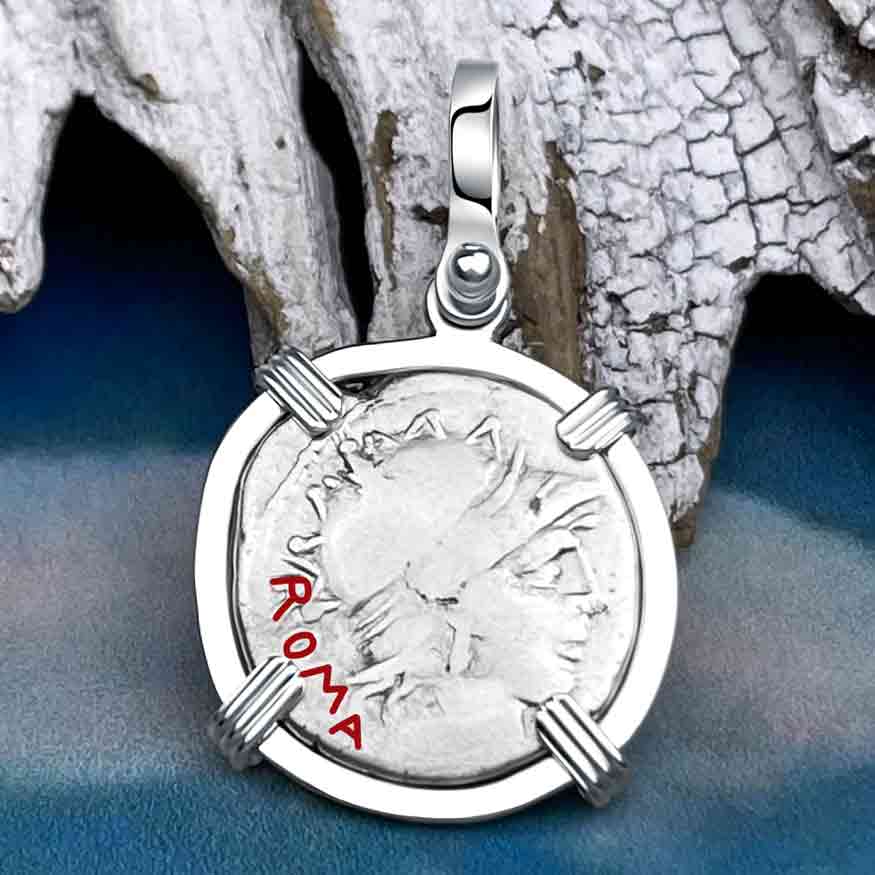This is a detailed photograph of a silver medallion, intricately designed to function as a pendant. The medallion showcases a well-worn Roman coin encased within a circular silver frame, secured by silver brackets positioned at the upper left, upper right, lower left, and lower right. A small, round joint attached to the top connects to an additional ring, allowing the medallion to be worn as a necklace. 

The coin itself displays the profile of a Roman emperor, helmeted and facing right, albeit with worn details that obscure some of the finer features. Prominently, the word "ROMA" is inscribed in red letters on the lower left part of the coin. 

The medallion is placed on a surface with shades of blue, and it is propped against a piece of driftwood, which exhibits variegated tones of white, brown, and silver, enhancing the rustic ambiance. The background appears to blend shades of dark blue, contributing to the overall artistic composition of the photograph.